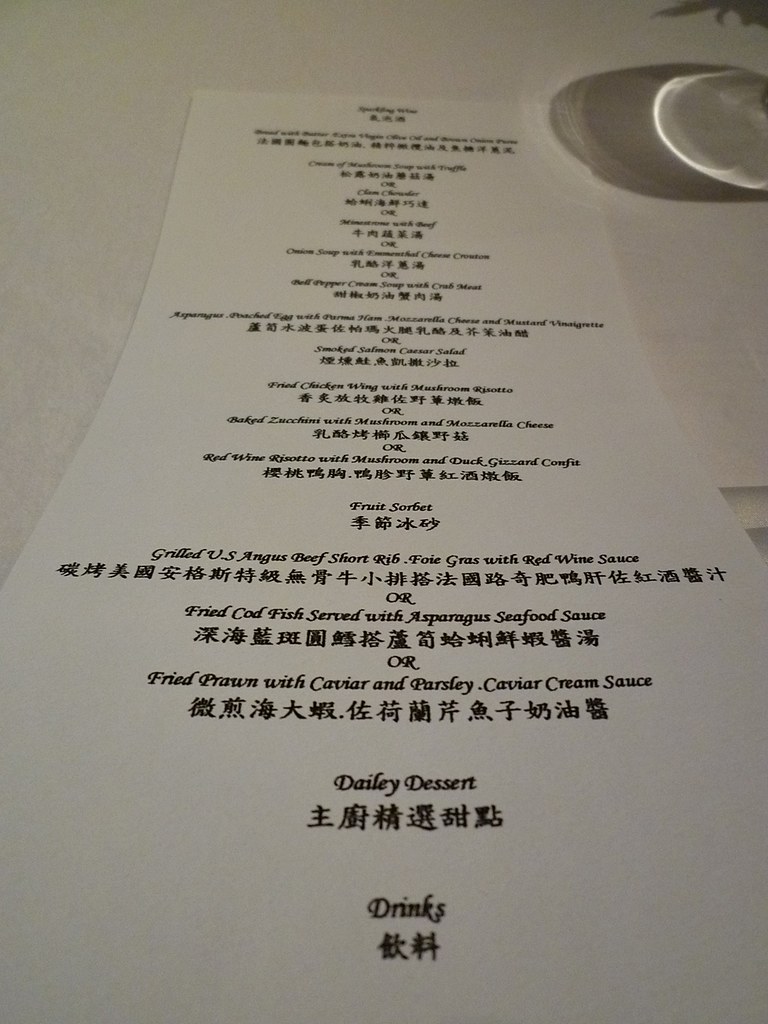This image captures a sleek, white table adorned with a lengthy, rectangular menu. The menu, primarily written in an elegant black typeface, displays text in both Asian characters and English. At the bottom of the menu, the word "drinks" is prominently visible, alongside phrases like "deli," "dessert," and "fried prawns," though some text is small and challenging to decipher. The menu items are listed with English descriptions first, followed by their Asian counterparts. To the right of the menu, a subtle shadow is cast, accompanied by the base of a glass or wine glass, adding a touch of sophistication to the scene.